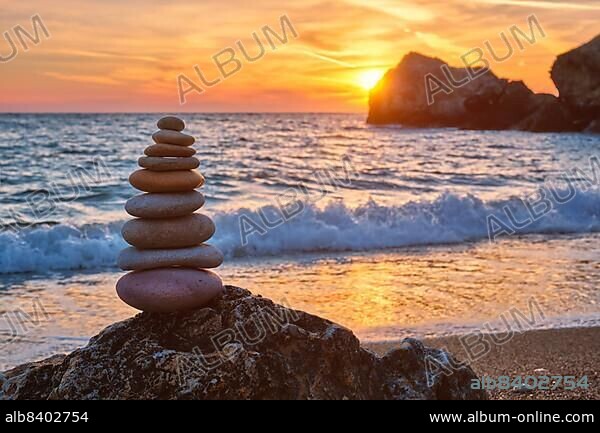The image captures a serene beach scene at sunset, with the sun setting behind a prominent rock outcropping in the ocean, casting a peachy pink-orange glow across the sky. In the immediate foreground on the left, there is a significant stack of nine flat rocks balanced on a larger rock, emphasizing a zen-like tranquility. Waves are seen crashing near this rock stack, with a frothy white wave rolling toward the shore and another receding wave moving back out to sea. The sandy beach is visible in the bottom right corner. The horizon is defined by a dark blue line in the distance, with scattered clouds enhancing the vividness of the sunset. The bottom left corner features a black border with the text "ALB 8402754," and the bottom right corner displays the website "www.album-online.com" along with the same text, "ALB 8402754."